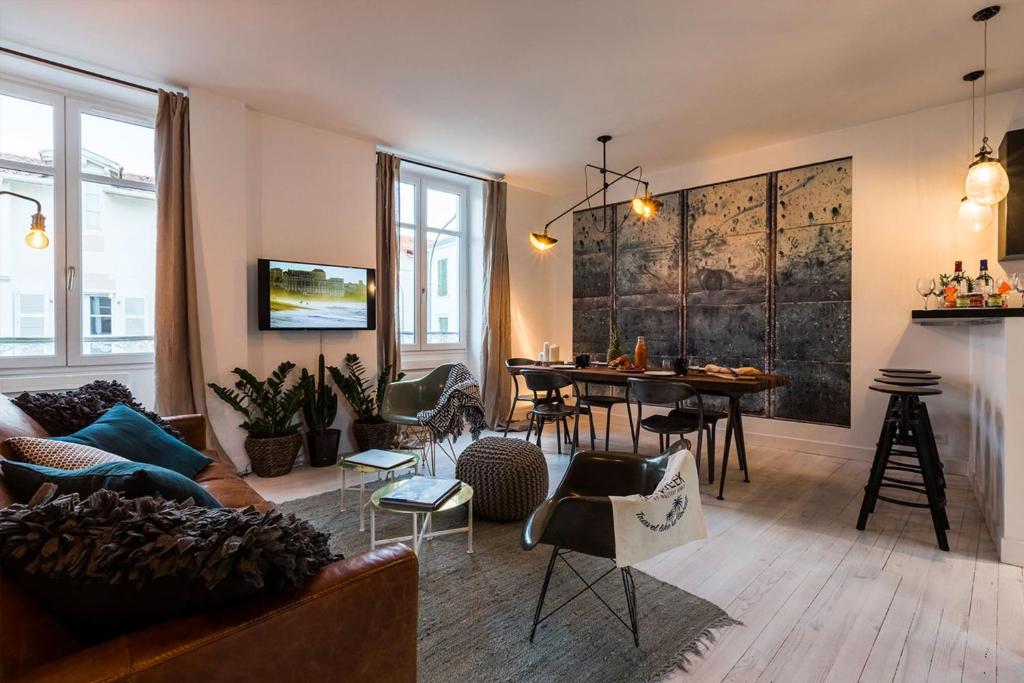The image captures a stylish and modern studio apartment with a seamlessly integrated living and dining area. The open space features sleek, light-colored flooring that resembles wood or possibly vinyl paneling with a warm sandalwood hue. The cream-colored walls are bathed in soft yellow lighting, giving the room a cozy, inviting ambiance. 

On the right, a kitchen counter with four bar stools leads into the dining area, where a long wooden dining table sits, surrounded by black steel chairs. Above the dining table, unique abstract art, split into multiple panes, decorates the back wall.

The living area boasts large, open windows with brown curtains that frame a mounted TV, below which three potted plants and a chic plastic chair with steel legs can be seen. The comfortable seating arrangement includes a large brown leather couch adorned with blue and furry brown pillows, various chairs, ottomans, and side tables, all anchored by an area rug that adds to the room’s welcoming feel.